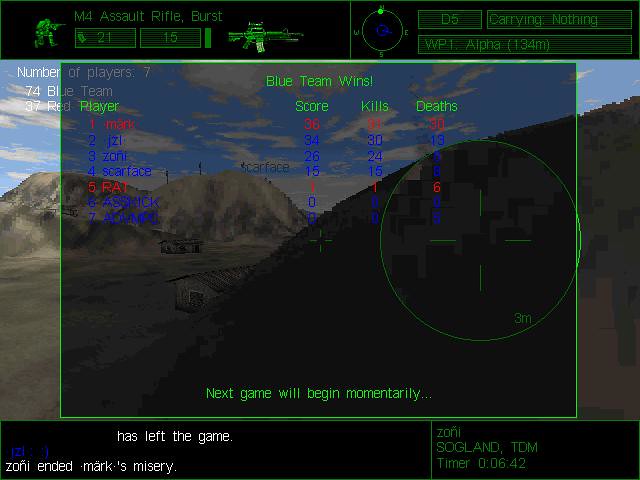In the center of the screen is a bee perched on a video game console, captured perfectly in the middle of the action. At the bottom left corner, the screen displays the names "Sohye" and "Mark Spicery." To the right, there is a game text indicating "Sohye Soglin, TDM," with a timer showing "0.0642." Centrally located on the screen is a detailed scoreboard. The upper left corner of the screen reveals the number of players, which is 7. The Blue team has 34 points while the Red team leads with 37 points. Player information is displayed in blue text, but it's somewhat obscured due to the background, listing up to two player names in a vertical stack. The scoreboard also details that the current match is based on scores, kills, and deaths, stating that the Blue team's score is 36 with 31 kills and 30 deaths, although the clarity of these numbers varies. The upper left also shows a player crouching, wielding an M4 assault rifle in burst mode, with ammunition counts appearing as "21," "15," and noting a "D5 Carbon."

This intricate amalgamation of active gameplay and interface details showcases a dynamic moment within the game, sprinkled with specifiable metadata and player statistics.